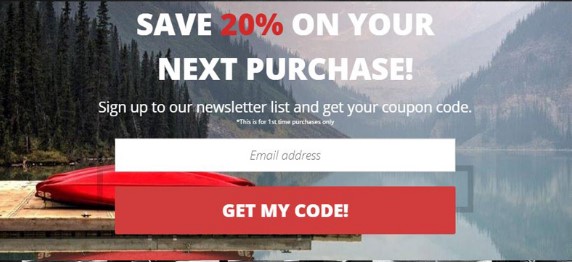"Discover the Great Outdoors with Our Exclusive Offer! Save 20% on your next purchase by signing up for our newsletter. Enter your email address and click the big red 'Get My Code' button to receive your coupon code. *Note: This offer is valid for first-time purchases only. The background showcases a serene lakeside scene with a picturesque view of majestic mountains and lush trees. A wooden pier stretches into the calm, reflective waters of the lake, where a red canoe rests upside down near the end, presumably drying out. The overcast sky lends a foggy ambiance, mirroring beautifully on the lake's surface. The '20%' discount is prominently displayed in bold red text, while the rest of the message is in white, inviting nature enthusiasts to seize this opportunity. Ideal for those who appreciate the tranquility and adventure of the great outdoors."